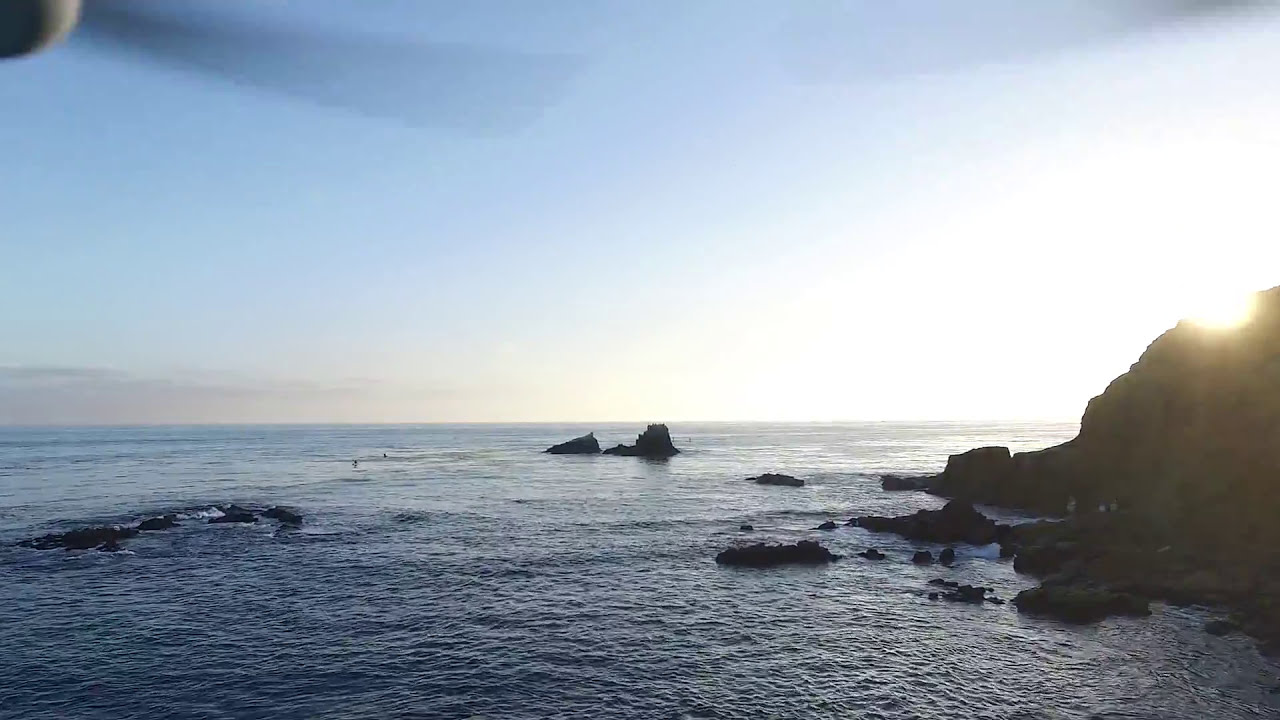This stunning aerial photograph, likely taken from a helicopter given the visible blurred rotor blades at the top of the image, captures a breathtaking ocean vista during sunset. The scene looks out over a calm yet dynamic expanse of ocean, dotted with rocks and boulders that the waves gently crash against. To the right, a jagged cliffside towers with the sun setting behind it, casting a golden glow that blends beautifully with the clear sky's blue and pink hues. Off in the distance, small flocks of birds add life to the serene image, and the calm waves suggest a tranquil moment captured high above this picturesque coastline.